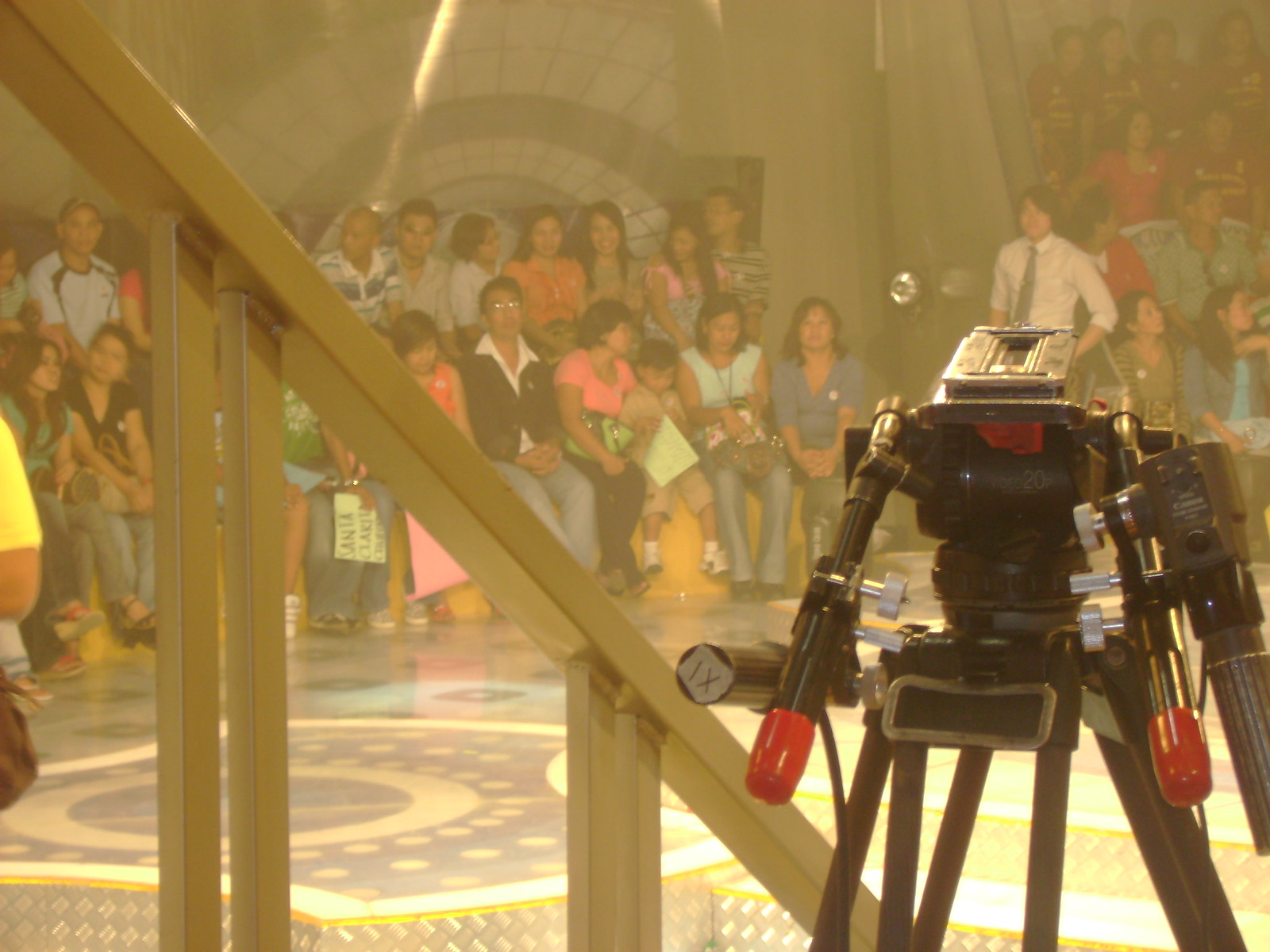The image captures a lively indoor gathering at a convention or museum, decorated ornately with a beige banister and a beautiful circular tile floor pattern. A diverse crowd, composed of several dozen people including many Asians, spans all ages from children to adults, and they are seated in rows on benches, creating a sense of anticipation as if waiting for a presentation or speaker. Many colors are noticeable in the scene—black, white, gray, brown, beige, pink, yellow, orange, red, and green. 

In the foreground, there is a black tripod with red knobs, possibly for a video camera, and a nearby robotic figure labeled "1X" with a "20" by its face—this robot is black with red arms and silver accents on its head and top part of its arms. The crowd is closely packed, with people appearing happy, engaged, and enjoying the moment. A young man stands out among the audience, dressed in a white button-down shirt and black tie, with his hands on his waist, possibly part of the event's crew. The scene is lively, with a potential TV program setup in the background, indicating a significant event is about to unfold.